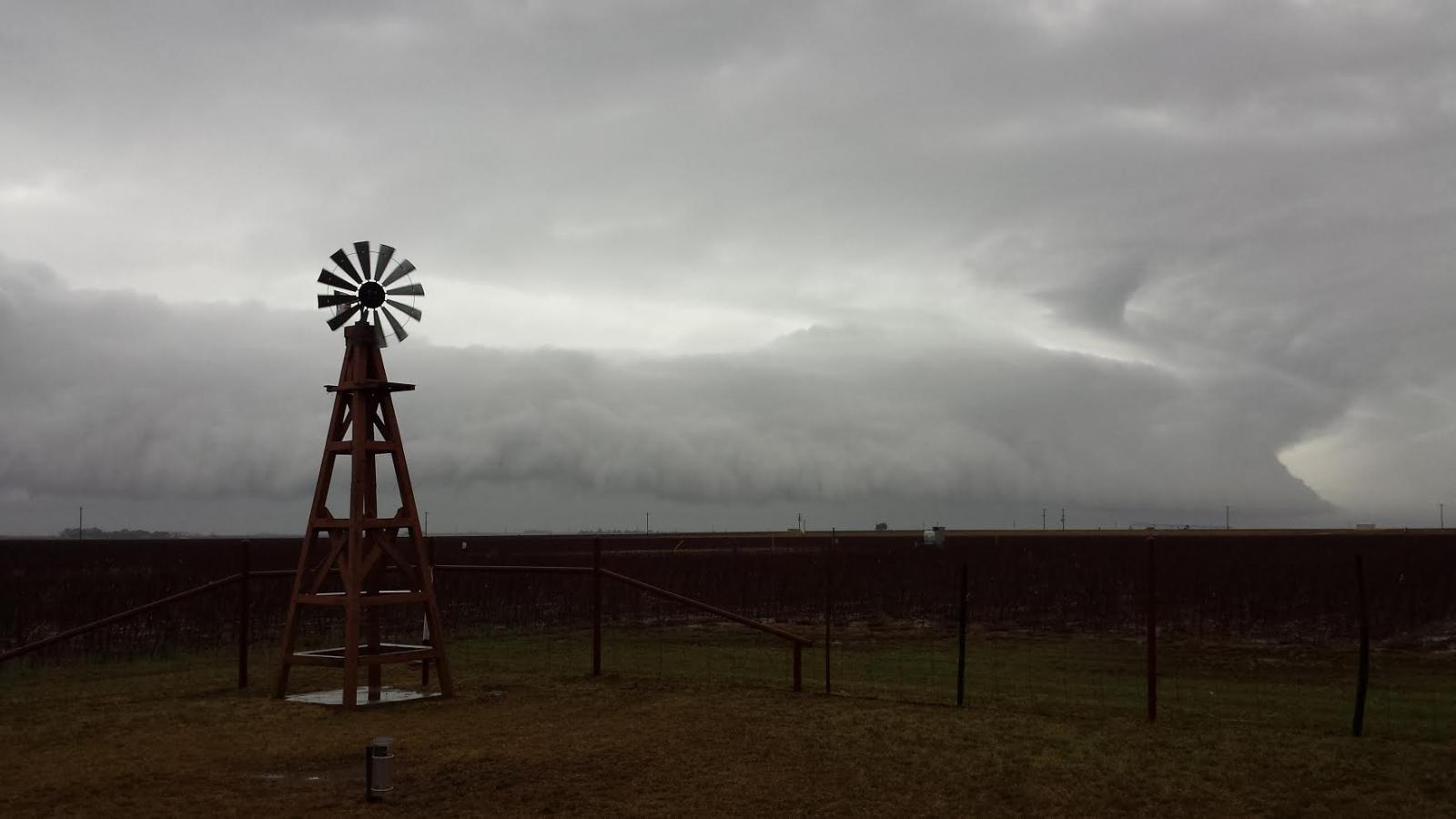The image depicts a dimly lit, almost black-and-white scene of a vast, open landscape under a stormy sky. Ominous, thick clouds, characteristic of an occluded front that can bring hail or tornadoes, dominate the horizon, casting a dark and foreboding atmosphere over the flat land, which could be somewhere like western Kansas or eastern Colorado. In the foreground, an aged wooden windmill stands tall, evoking a sense of bygone days with its triangular structure and wheel-like blades at the top. This windmill is typically associated with a water-pumping mechanism, although no tank is visible in the image. Surrounding the windmill is a dirt-covered ground transitioning to patches of greenish, yellowish grass. A fence, composed of dark-colored posts and likely wires, forms a perimeter around the windmill area. Despite the poor lighting, the photograph captures the contrast between the stormy sky and the flat, expansive terrain below, highlighting the dramatic and impending weather.